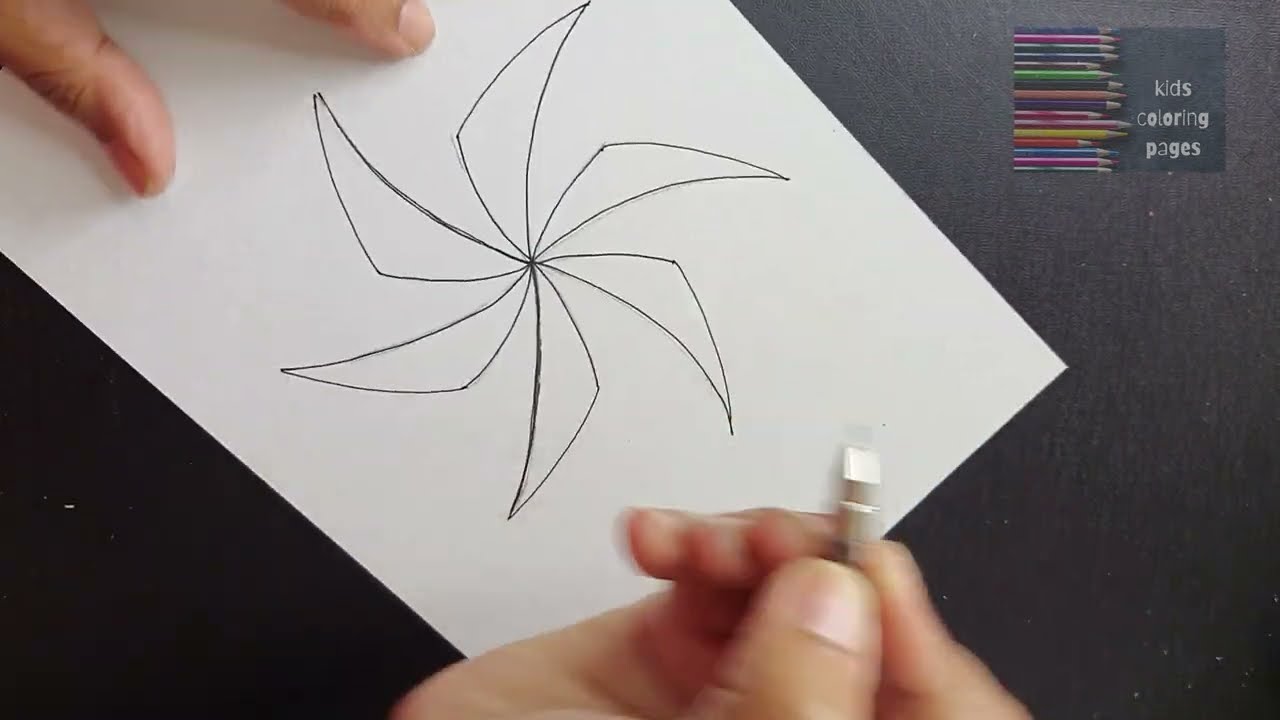The image captures an overhead view of an artist in the process of drawing a windmill, specifically focusing on the arms of the windmill that form a pinwheel-like shape with six curved petals or triangles. The intricate design is rendered in pencil on a white piece of paper, which is set diagonally on a black, grainy, textured surface. The artist's fingers are visible, with the right hand caught in motion, holding a silver pen, and the left hand stabilizing the paper. In the upper right corner of the image, there is a semi-transparent blue rectangle containing various colored pencils arranged horizontally, accompanied by three lines of white text that read "Kids Coloring Pages."